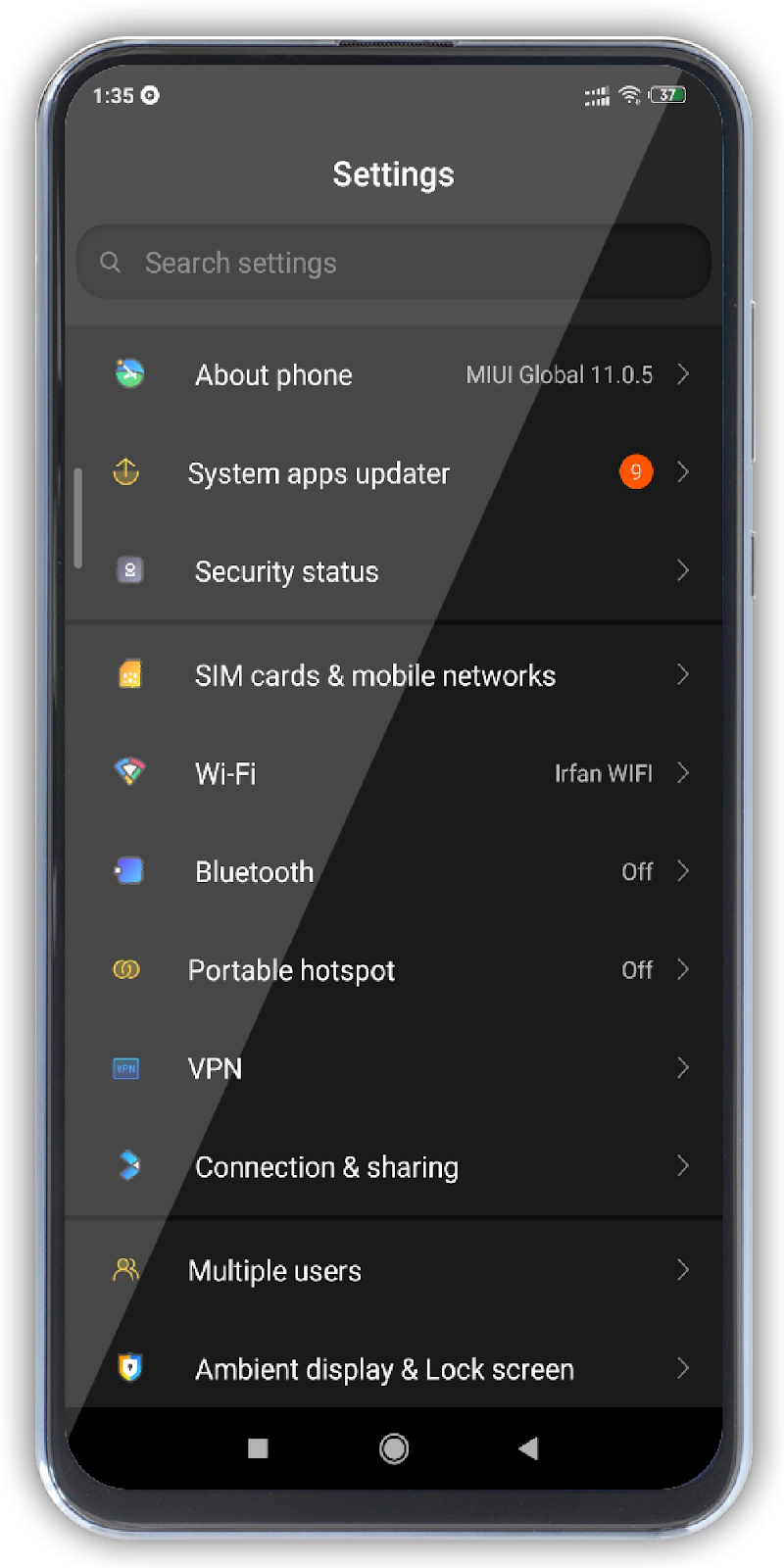The image is a detailed screenshot of the settings page on a Xiaomi mobile phone. The phone itself features a sleek silver outline around the edge, contributing to its refined appearance. The screen showcases a predominantly black background, with a distinct shadow gradient extending from the upper right-hand corner to the lower left-hand corner, giving a contrast between the sunlit top half and the shadowed bottom half.

In the top left corner of the screen, the time is displayed as 1:36, accompanied by a circular icon. On the top right corner, status icons for Wi-Fi and battery are visible. Centrally placed on the screen is the word "Settings" in white text, followed by a greyed-out search bar labeled "Search settings."

Below the search bar, there is a list of various options, each paired with small colorful icons on the left. The options visible include "About phone" and "Systems app updates," the latter marked with a red circle. Other listed settings include "Security status," "SIM card & mobile networks," "Wi-Fi," "Bluetooth," "Portable hotspot," "VPN," "Connections & sharing," "Multiple users," "Ambient display," and "Lock screen," each accompanied by directional arrows indicating further sub-menu options.

"Wi-Fi" is connected, showing "Irfan Wi-Fi," while both "Bluetooth" and "Portable hotspot" are turned off. At the screen's bottom, navigation icons are displayed: a square-shaped button on the left, a round button in the center, and a back button on the right.